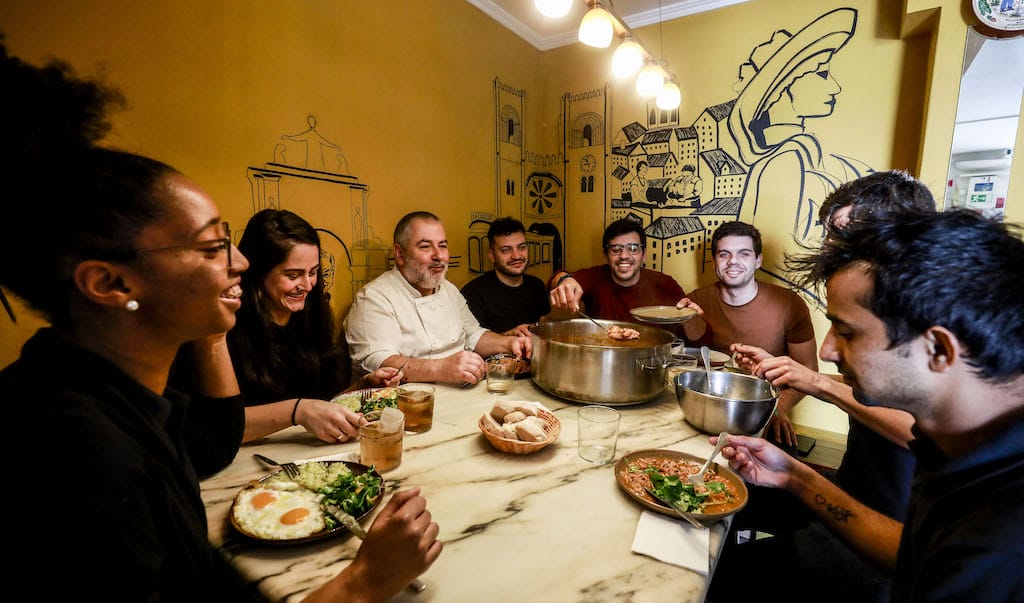In the image, a group of friends or family are gathered around a large, white and black marble-topped table, enjoying a meal together. There are eight people in total, a mix of different genders and ages, all dressed in various colors such as green, white, orange, black, yellow, brown, and red. On the table, there’s an assortment of food and drink: one person is eating eggs and greens while another is seen with beans. A silver pot, likely containing seafood, stands prominently in the center, with one person scooping food from it, complemented by a smaller silver bowl being used by another. Also featured on the table is a basket of bread and glasses filled with drinks.

Surrounding them are mustard-yellow walls adorned with a mural depicting the silhouette of a woman and village buildings, rendered in a stenciled black design. The lively ambiance is highlighted by overhead lights, and everyone appears to be enjoying themselves, immersed in the pleasant atmosphere of the scene.